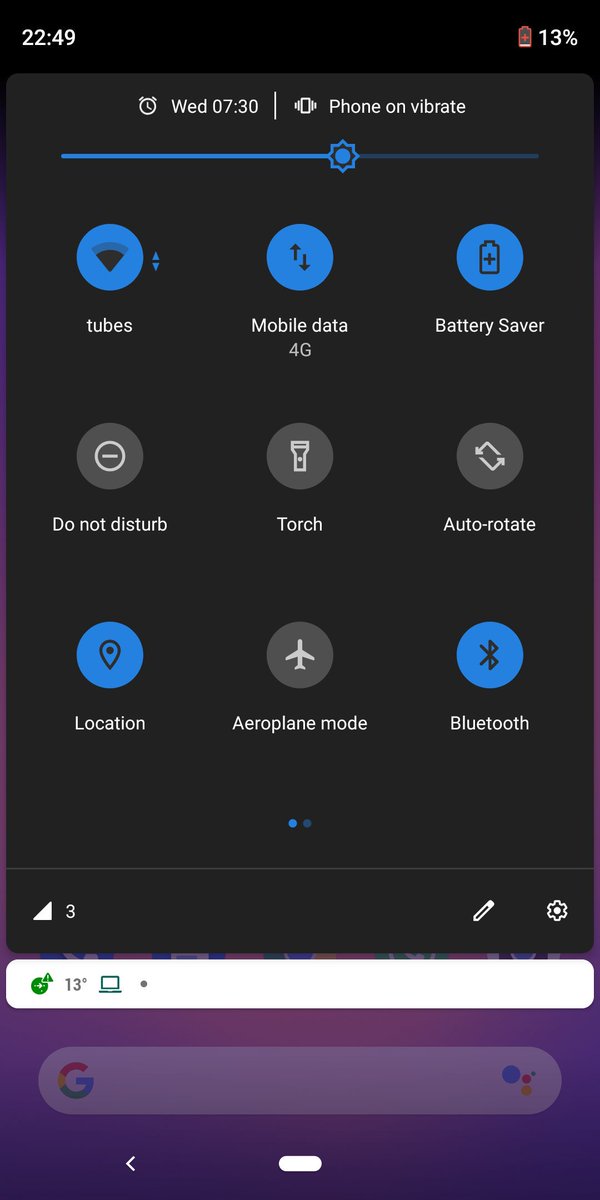The image showcases a smartphone screen with various interface elements and system notifications, reflecting a specific state of device usage and settings.

At the top of the screen, the digital clock displays the time as 22:49, and the battery icon indicates 13% remaining battery life. Adjacent to the time, there's a small clock icon followed by the text "Wednesday 7:30," indicating an upcoming alarm. The phone status is also shown, indicating that it is set to vibrate mode.

Beneath these notifications, there is a volume bar. The bar appears predominantly dark blue, showing the current volume level, which is above halfway, while the remainder of the bar is in a grayed-out blue, representing the inactive portion.

Further down, a series of toggles for quick settings are displayed. The first set includes:
- "Tubes"
- "Mobile Data 4G"
- "Battery Saver"

These toggles appear to be active, indicated by their blue color.

Below these, there are additional quick settings toggles:
- "Do Not Disturb"
- "Torch"
- "Auto Rotate"

These, however, are inactive and displayed in a gray color.

The final row of toggles includes:
- "Location" (active and blue)
- "Airplane Mode" (inactive and gray)
- "Bluetooth" (active and blue)

At the very bottom of the screen is a white bar displaying the number "13" next to a small laptop icon, likely indicating a device connection or battery-related information. Below this bar is the familiar Google search bar, providing quick access to the internet search function.

This detailed configuration snapshot offers a comprehensive view of the user’s phone settings and operational status at the given moment.